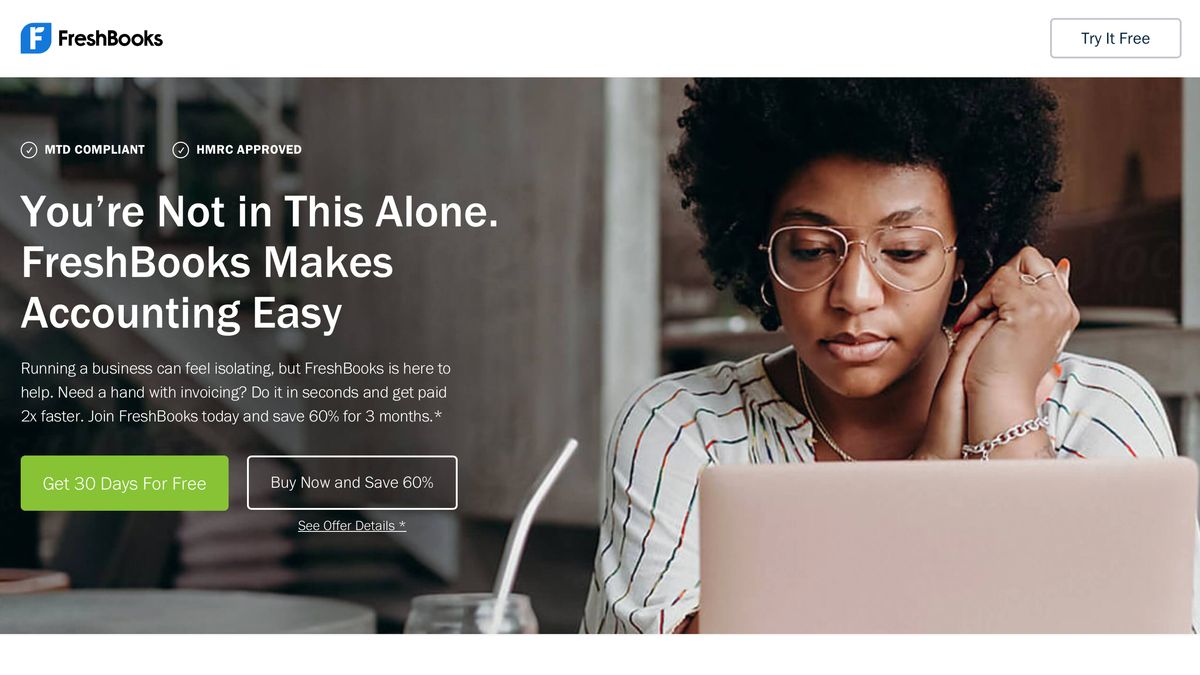The image features the homepage of the FreshBooks website. In the upper left corner, the FreshBooks logo is displayed, consisting of a blue leaf with a white 'F' inside it, followed by the company name in black text. To the right of the logo, there's a call-to-action button that says "Try it Free," which is white with a black outline and black text.

Below, there's a photograph of a woman working on a laptop. She is positioned on the right side of the image, while the left side shows her room in the background. She is using a light pink laptop, with its screen open, focusing intently on her work. The woman, a Black female, has a large afro and wears aviator glasses. Her fingernails appear to be painted orange.

To the left of the woman, text reads "MTD compliant, HMRC approved," each statement accompanied by a small circle with a check mark. Below this, in large white capital letters except for the letter 'N', the text states: "YOU're NOT IN THIS ALONE. FreshBooks MAKES ACCOUNTING EASY." Further down, in smaller white font, the text continues: "Running a business can feel isolating but FreshBooks is here to help. Need a hand with invoicing? Do it in seconds and get paid two times faster. Join FreshBooks today and save 60% for three months."